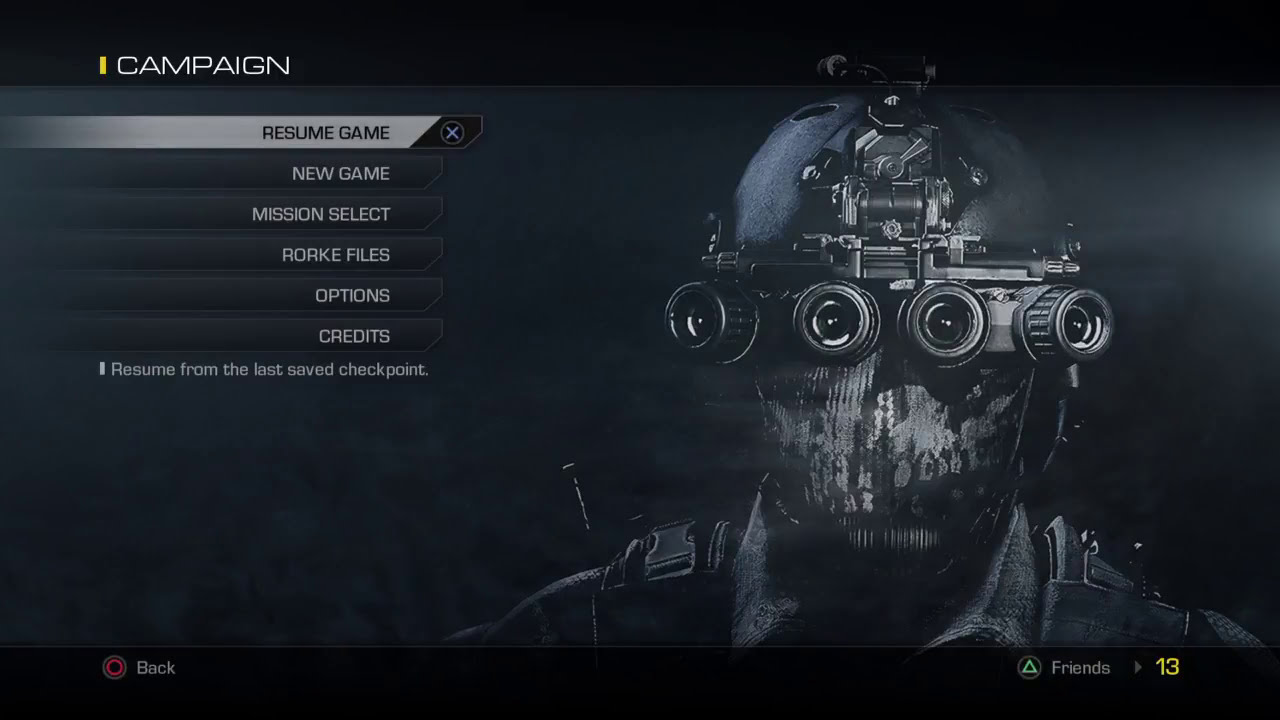The image captures a screenshot of a video game's campaign menu. At the top, "Campaign" is displayed in white text, followed by a series of options: "Resume Game," "New Game," "Mission Select," "RORC Files," "Options," and "Credits." Below these options, it specifically mentions "Resume from last saved checkpoint" in smaller text. The layout features black borders at the top and bottom, giving the background a smoky gray appearance. In the bottom left corner, there's a red circle button labeled "back," while the bottom right corner has a green triangle button labeled "friends" with the number 13 in yellow. Dominating the right side of the screen is a futuristic, militaristic character. This character is adorned in high-tech gear, including a black helmet, night vision goggles with multiple lenses resembling eyes, and a mask that covers his entire face. He wears a black collared shirt with various straps over his shoulders, possibly indicating a tactical vest. The lighting highlights different parts of his helmet, creating a subtle shine.